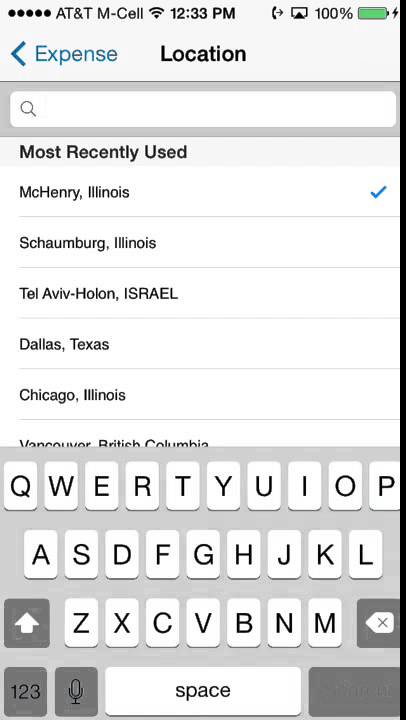This is a meticulously organized screenshot of a smartphone interface displaying location-based data. At the top of the screen, the title "Location" is prominently featured in bold black text. To the left, a blue header labeled "Expense" is accompanied by a blue back button, allowing for easy navigation. Below this, a white search bar set against a gray background provides a space for users to input their queries.

Beneath the search bar, the section titled "Most recently used" is showcased, indicating the most recent locations selected. The list begins with "McHenry, Illinois," highlighted with a blue check mark, signifying it as the chosen location. Following this, a series of other locations are displayed, each separated by thin gray lines for clarity. The list includes Schaumburg, Illinois; Tel Aviv; Holon, Israel; Dallas, Texas; Chicago, Illinois; and Vancouver, British Columbia.

At the bottom of the screen, the pop-up phone keyboard is visible. The keyboard features a gray background and white keys, ensuring a clean and functional user interface. The overall background of the screen is white, maintaining a cohesive and uncluttered design.

Additional details include crucial information at the very top of the screen: the battery is fully charged at 100%, as indicated on the top right. On the top left, the cellular carrier is identified as AT&T. Centrally positioned between these two indicators, the current time is clearly shown as 12:33 p.m.